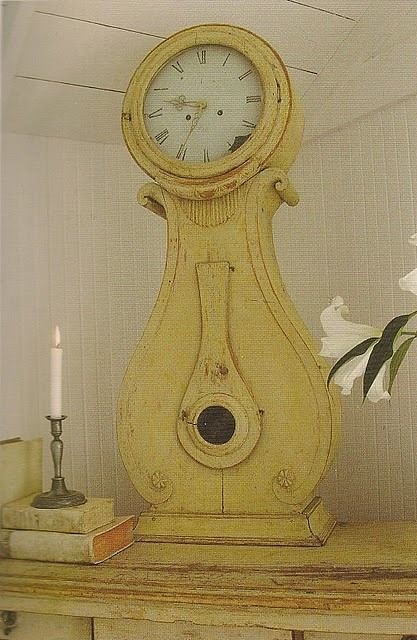This is a highly realistic, vertical, and rectangular color painting of an extremely tall and thin vintage clock on a mantelpiece. The scene is set in what appears to be the corner of a room with Scandinavian-style décor, characterized by white wooden walls with vertical lines and a white wooden ceiling with thicker horizontal pieces. The clock, made of yellow-tinted wood, features a unique design. At the top is a round clock face with gold, intricately designed, steampunk-style hands pointing to 9:35, and Roman numerals decorating the dial. The wooden structure beneath the clock face showcases a carved shape resembling a lute or harp, and it rests on a rectangular base with small, scroll-like details and a dark circular accent near its bottom.

To the left of the clock sit two old-style books with a lit white candle on top, held in a pewter candlestick. To the right, one can see a calla lily and part of another, enhancing the serene ambiance of the scene. The mantelpiece, matching the yellow-tinted wood of the clock, is adorned with a lighter strip of wood underneath, adding to the aesthetic appeal of the composition.